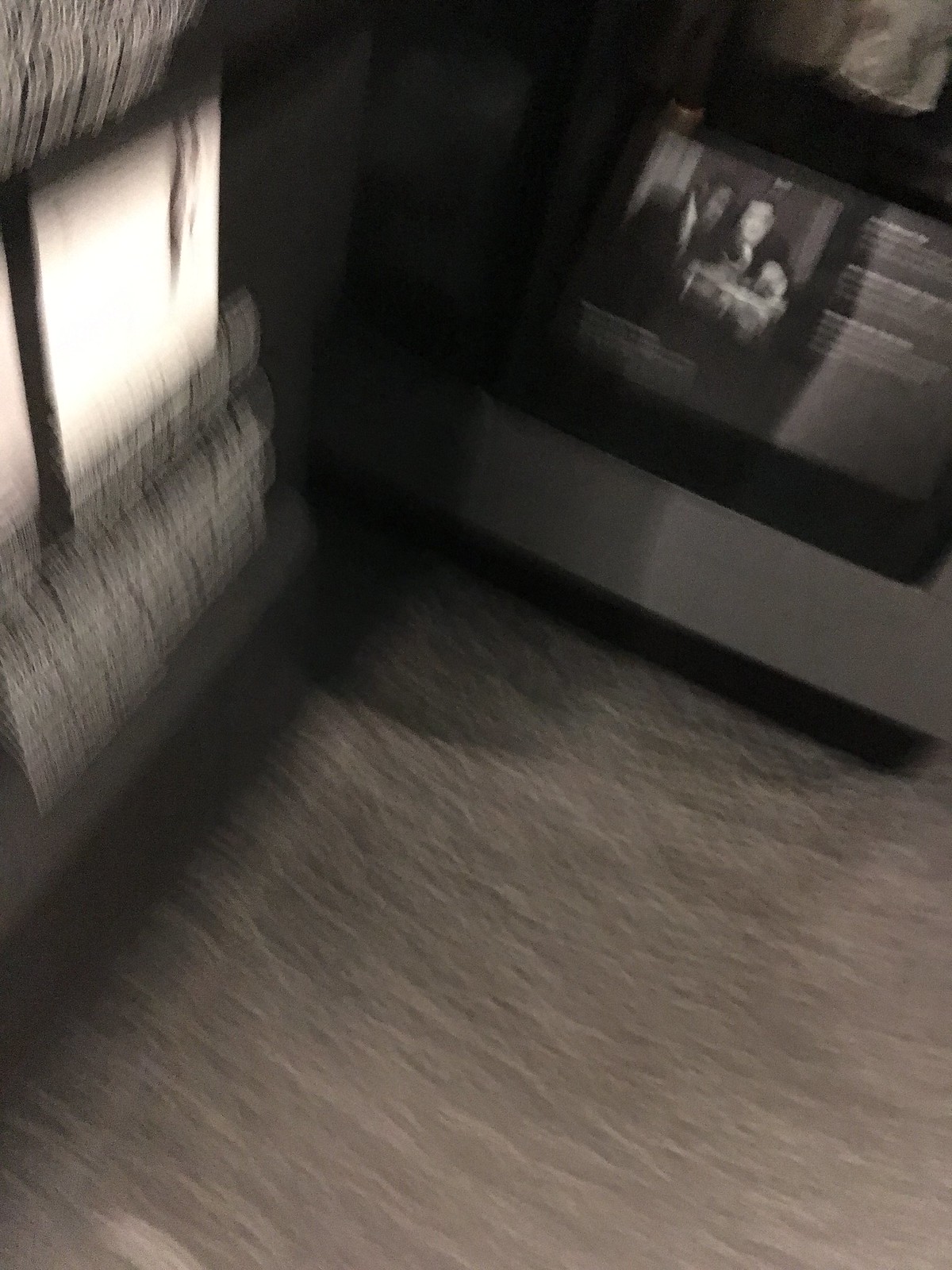This photograph is quite blurry and out of focus, predominantly displaying various shades of gray. The most discernible element is a black-and-white television located in the top right-hand corner of the image. The TV appears to be at an angle, requiring a head tilt to the right for proper viewing. The screen seems to display a scene reminiscent of an old TV show, potentially "Perry Mason," featuring a white individual on the right and a black individual on the left side of the screen.

A large section of the photo is composed of a lighter gray, almost white, band running horizontally in the middle. This band divides darker gray-black areas at the top and bottom, suggesting a layered composition. To the left, there appears to be something resembling a white window, though it is not entirely clear. The overall image is hazy, with the television being the only recognizable element amidst the indistinct surroundings.